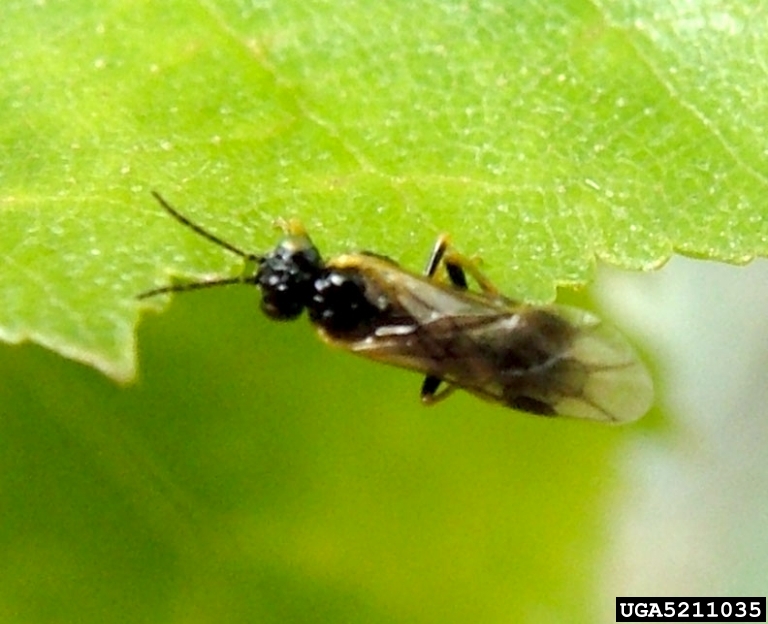The photograph captures a detailed view of an insect resting on a dark green leaf, which is veined with various shades of light green. The insect, which appears to be some type of fly, has a long, oblong black body, with six legs—three on each side. Positioned towards the top left corner of the image are its large head and two prominent eyes. Small antennae protrude from the top of its head. The insect's semi-transparent wings are a mix of clear, yellow, and black, and they are resting along its back. The leaf below it appears textured with a glossy sheen and scalloped edges. In the bottom right corner of the photograph, a black rectangle with white text reads "UGA 5211035."